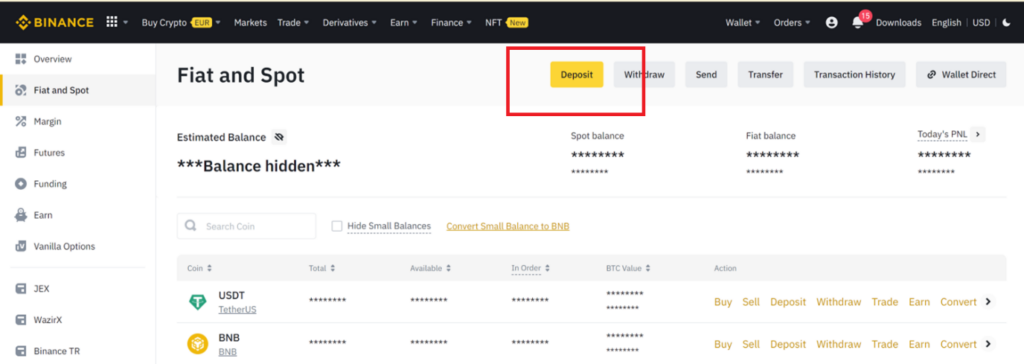This image appears to be a screenshot of the Binance website, specifically showcasing a user's dashboard interface.

At the very top of the screenshot, there's a black banner stretching across the width of the screen. On the far left side of this banner is the Binance company logo, followed by the text "Binance" and what seems to be an icon consisting of multiple dots. Adjacent to this, there are seven tabs available for navigation, though their text is too small to discern clearly. Two of these tabs are marked with yellow indicators, possibly denoting new features.

Moving to the right side of the black banner, several more icons and menu options are visible. One notable icon resembles an alert bell with a red notification badge in its upper-right corner, though specific details remain unreadable.

Beneath this black banner, a slimmer column on the left-hand side contains vertical navigation options. These options include sections labeled as "Overview," "Spot," "Margin," "Futures," "Funding," and "Earn," with several other unreadable entries. This left column is interspersed with thin gray dividers.

At the top of the main content area, there's a thin gray banner with the text "Fiat and Spot," under which lay five gray buttons extending towards the right. These buttons are labeled "Deposit" (highlighted in yellow and circled in red), "Withdraw," "Send," "Transfer," and "Transaction History."

Below these buttons, an "Estimated Balance" section is displayed, with the actual balance concealed by three asterisks (***Balance Hidden***). Adjacent to this are categories like "Spot Balance," "Fiat Balance," and "Today's Something," each accompanied by rows of asterisks implying hidden details.

Towards the right side of the interface, there’s a small search tab flanked by a checkbox and some light yellow text. Beneath this section lies another gray banner, organizing various columns which include filters or sorting options, though these column headings are too small to identify clearly.

Finally, the lower section features two prominent options for USDT and BNP, each represented by an icon on the left and followed by rows of asterisks, indicating private data. These options also have actionable buttons on the far right, although specific labels remain unclear.